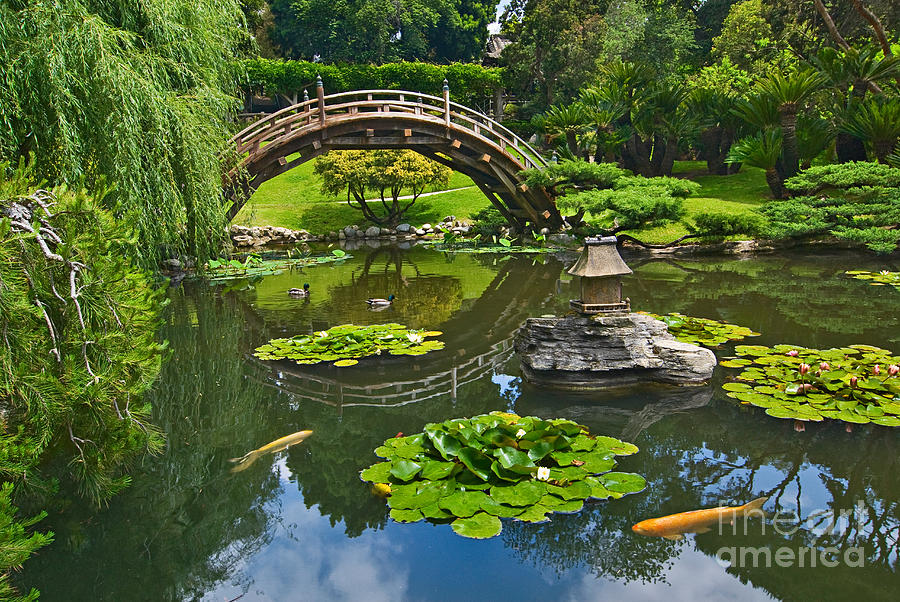The photograph captures a serene park scene centered around a picturesque pond. To the left, majestic Weeping Willows cascade their branches towards the water. The focal point is a charming wooden bridge with an arching, hilly shape, gracefully spanning the pond. The water is dotted with clusters of lily pads and vibrant, giant orange koi fish swimming beneath the surface. In the middle of the pond, on a cluster of rocks, stands a decorative birdhouse-like structure. 

The pond is teeming with life, as mallards float serenely alongside the lily pads. Surrounding the pond is a verdant landscape enriched with various trees, including bonsai-like shrubs and bright green trees that offer a canopy of shade. The grass fields stretch out into the distance, interspersed with short bushes and rocky formations at the water's edge. Benches are visible in the background, inviting visitors to sit and enjoy the tranquil setting.

The scene is bathed in daylight, with the bright blue sky peeking through the trees and the sun casting reflections on the water, enhancing the lush greenery and natural beauty of the park. The overall impression is one of peacefulness and natural elegance, capturing the essence of a sunny day in a well-tended park.